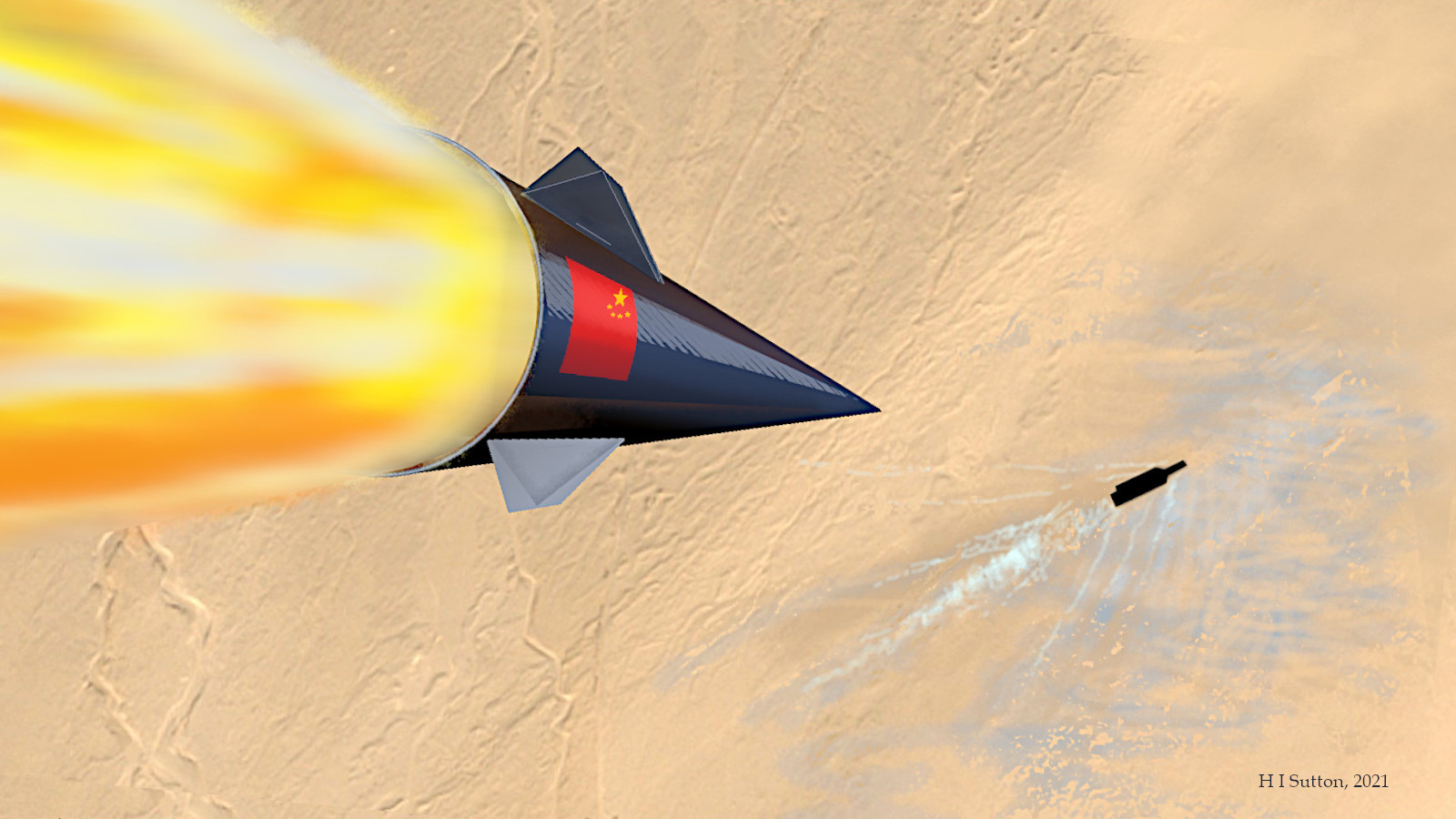The image is an animated, cartoonish drawing depicting a desert-like landscape with a tan, cracked ground and faint blue water spots to the right. From the top left corner, a blue, cone-shaped missile with the Chinese flag on its side is descending towards the Earth, expelling orange and yellow flames from its rear. The smooth, shiny surface of the missile reflects light, and it has two wings. In the bottom right corner, a black object, resembling a bomb or wine bottle, appears to have already been dropped. The scene includes a shadow at the bottom, suggesting the missile is about to crash land. The image is watermarked with "H.I. Sutton, 2021" in black text in the bottom right corner.